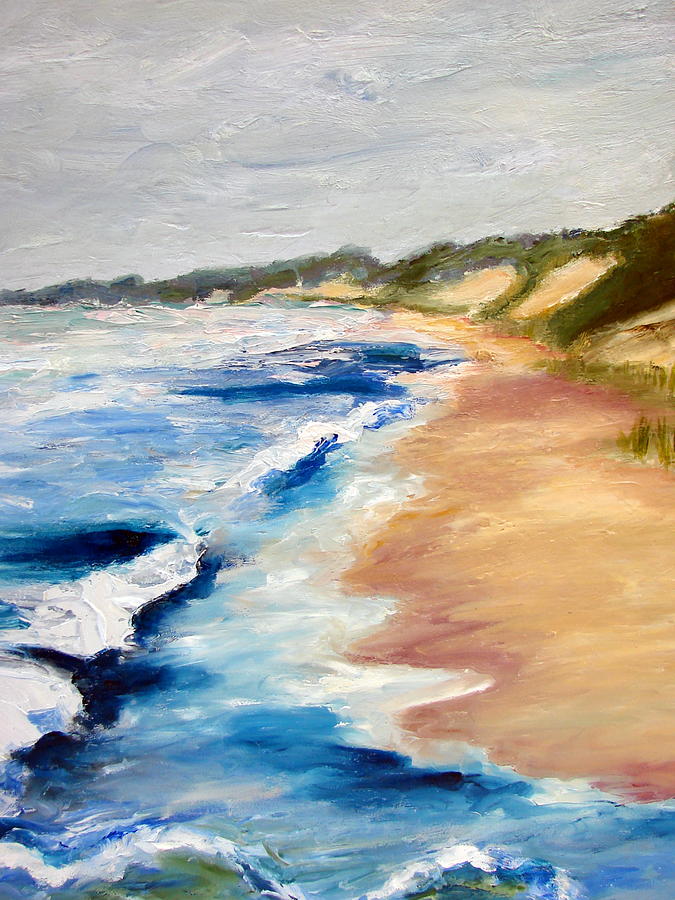In this detailed and evocative impressionistic painting, a tranquil yet stormy beach scene unfolds. The main focus is the blue ocean water, with waves lapping and crashing against a brown sandy shoreline situated on the right side of the image. The water is a rich royal blue, emphasizing its clarity and calm amidst the chaotic waves. The sandy beach transitions into green dunes adorned with grass and plants, curving gently toward the back of the scene. Overhead, a dramatic gray sky filled with textured, brush-stroked clouds enhances the impending storm atmosphere. The waves, capped with white foam, add dynamic movement to the serene, yet tumultuous, coastal landscape. This simple but powerful painting captures the unpredictable essence of nature, blending calmness with the beauty and force of the natural world.